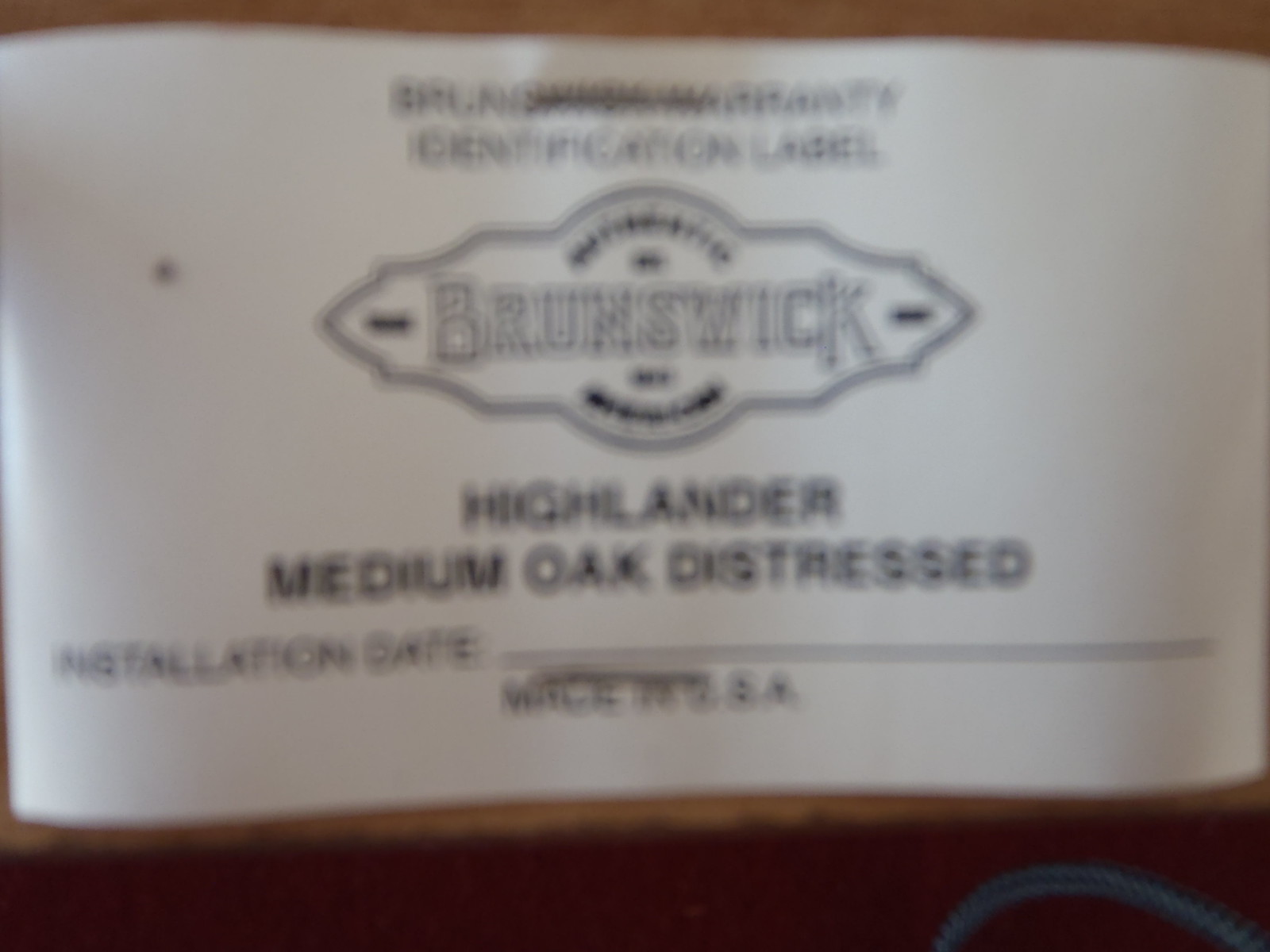This image features a rectangular tag or product label that is slightly out of focus, making the text challenging to read. The tag itself is primarily white and rectangular, with hints of red or dark brown near the bottom, accompanied by a curved, dark gray shape whose purpose is unclear.

The tag contains several lines of black text. At the top, a line of text is present but not legible. Below this, the text "Identification Label" is visible. Positioned centrally on the tag is a logo with an irregular shape, above which the word "Brunswick" is prominently displayed in larger text. Additional text is situated both above and below "Brunswick," though it remains indecipherable.

Further down the tag, the text reads "Highlander Medium Oak Distressed," followed by the label "Installation Date" and a blank line intended for recording the date of installation, which remains unfilled.